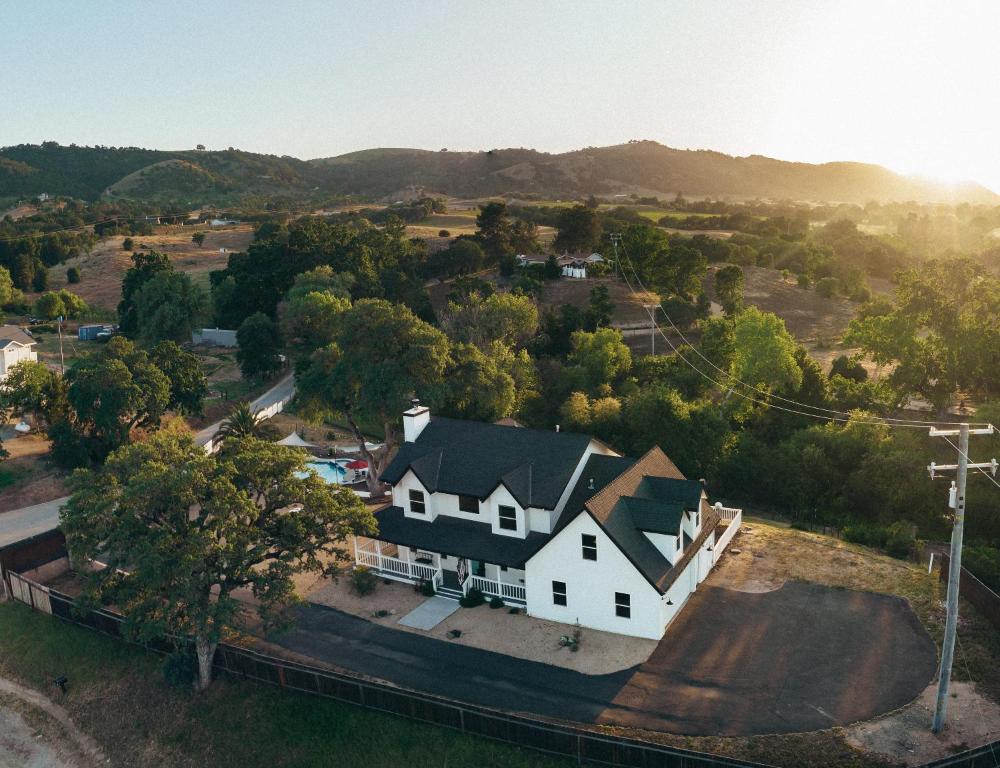The aerial photo captures a picturesque suburban home set in a tranquil environment. The primary focus is a two-story white house with a black roof and an attached garage with a second story. The house is enclosed by a fence and has a small pool in the backyard. A large tree stands prominently in the bottom left corner of the property, with a palm tree also visible in the backyard, indicating a climate where palm trees can thrive.

Beyond the fenced yard, a dense forest extends from one side of the photo to the other, creating a natural backdrop that scatters into individual trees further in the distance. Nestled among the trees are a few other homes, suggesting a semi-rural neighborhood. In the far background, rolling hills rise gently, with the sun just above the horizon on the far right, casting a warm glow over the landscape. Additionally, a small town road can be seen on the left side of the image, moving towards the center, with power lines stretching along it. This richly detailed scene beautifully blends elements of suburban life with serene natural surroundings.